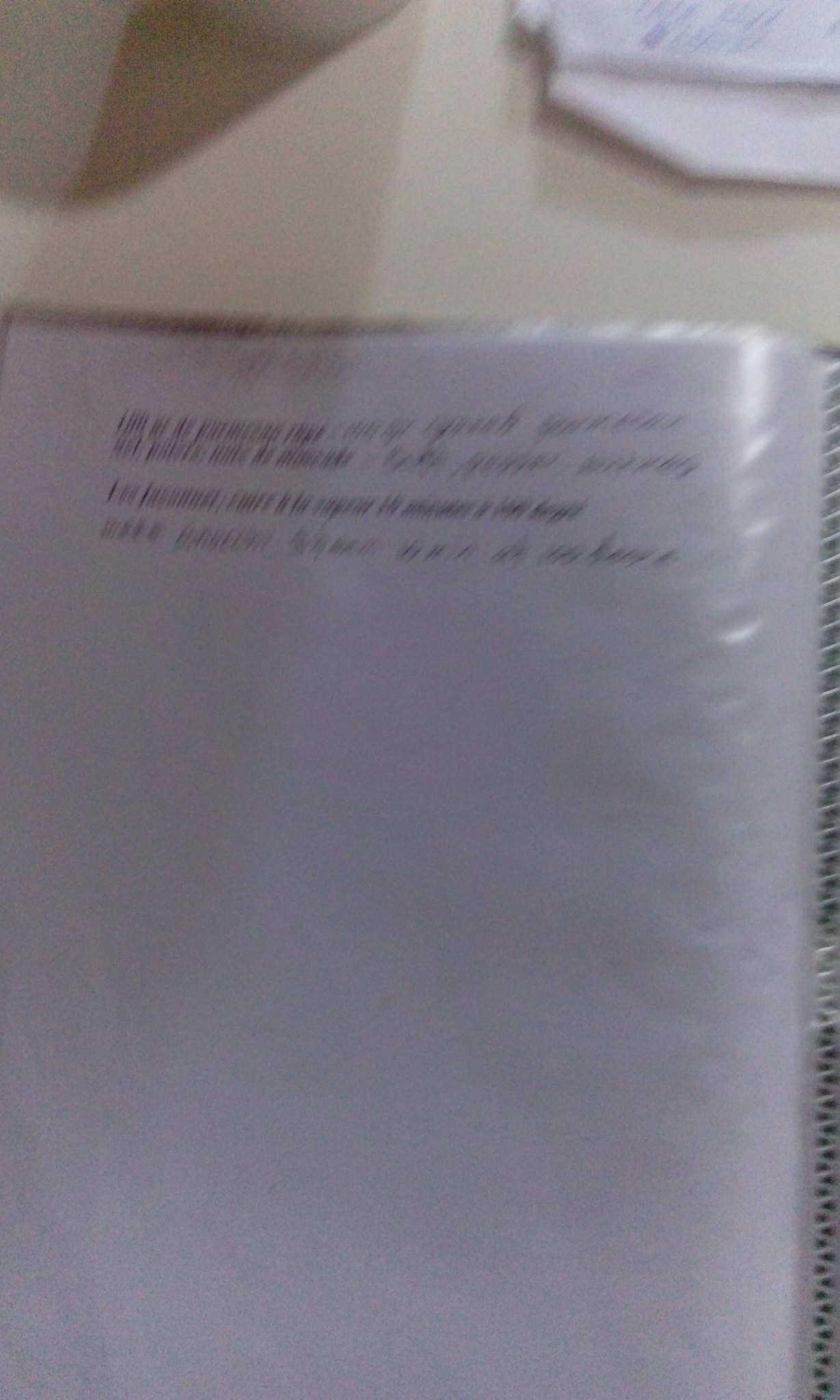The image is a blurry photograph featuring a completely unopened bar of soap, wrapped in transparent plastic with a paper label still intact. The soap is an off-white color and has unreadable writing across it, possibly in Chinese, which is obscured due to the blur. The photo is taken from a top-down perspective, showing the bar of soap placed on a beige or taupe-colored surface. Above the soap, there is an off-white shelf with what appears to be folded towels or shirts and some white material with blue accents on it. Light is shining down from the top of the image, casting shadows and adding to the overall blur of the scene.